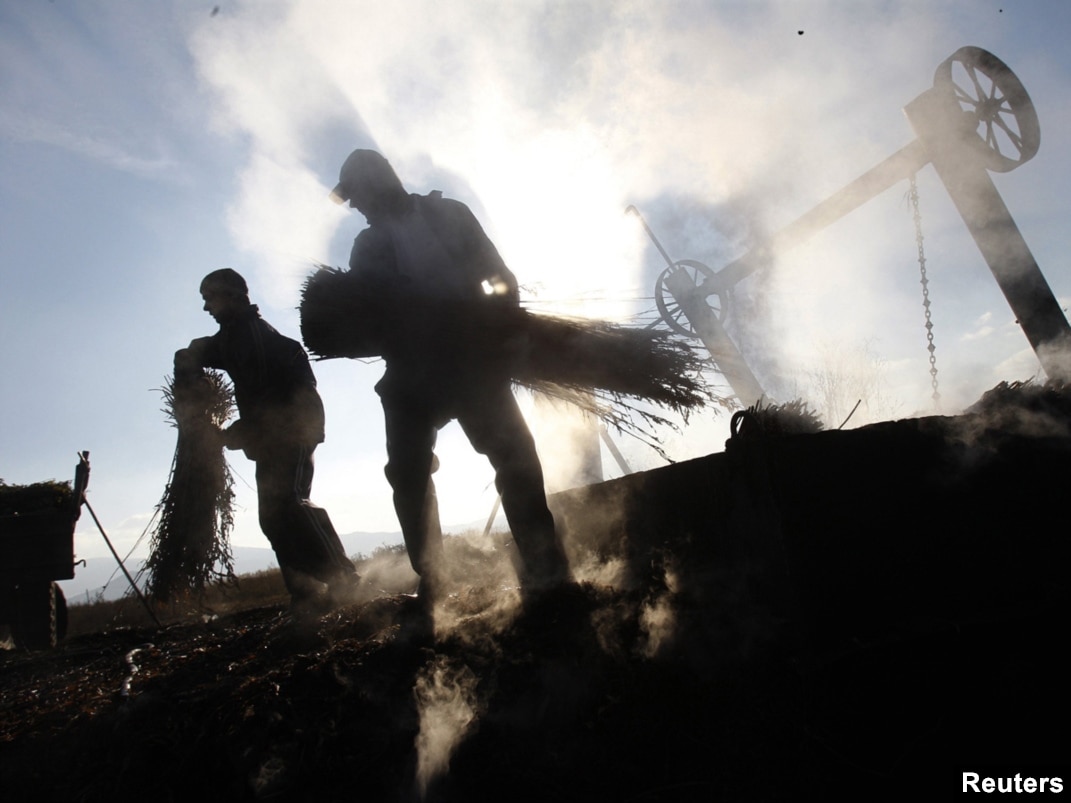This Reuters photograph captures a dramatic scene of two silhouetted men working in a field under a blue sky with wisps of clouds and rising dust or smoke. Taken during the day, the image is steeped in shadows, rendering the figures almost entirely black and devoid of discernible features. The man on the left, seen in profile and wearing a hat, and the man to his right, possibly wearing a beanie and a jacket, each hold large sheaves of wheat or barley. To the right stands a large vintage or antique piece of agricultural machinery, possibly a harvester, characterized by its prominent metal arms, large spoked wheels, and dangling chains. The dark, shadowy ground contrasts starkly with the lighter, slightly grayish blue sky, enhancing the silhouette effect. The bottom right corner of the image is marked with "Reuters" in white letters, signifying its source.